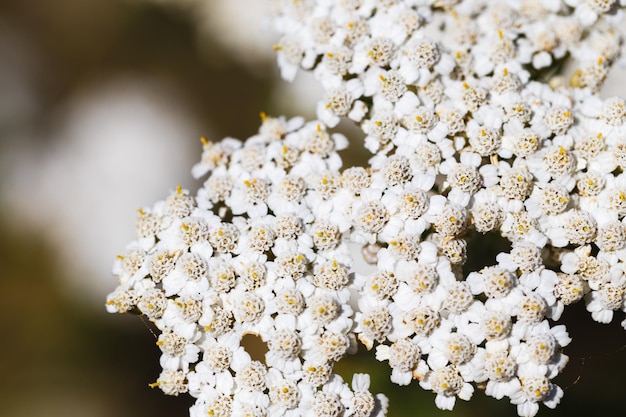The close-up image captures an abundance of tiny white flowers with a central yellowish structure, resembling cherry blossoms or poppy seeds. These delicate flowers are densely packed together, creating a solid expanse of white with each flower's intricate stamen visible. The soft overcast light enhances their snowy appearance, making them appear almost like popcorn scattered across the scene. The background is a blurred mix of greenish-brown hues with occasional white spots due to the camera's aperture, rendering the flowers as the sharp, unmistakable focal point. The lack of any greenery adds to the striking, almost surreal effect of the concentrated floral mass.